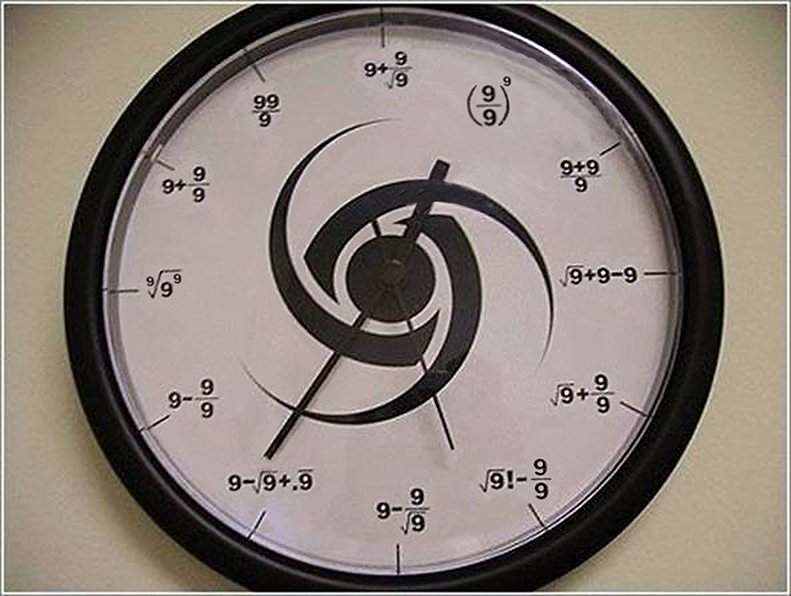This image portrays a uniquely designed clock where each numeral is replaced by a mathematical equation involving the number 9. The clock face creatively integrates various mathematical expressions to represent standard clock numbers. For instance, the number 1 is depicted as 9 divided by 9 to the power of 9, simplifying to 1. Similarly, the number 2 is represented by the equation 9 plus 9 divided by 2. Every numeral on the clock face is a clever mathematical arrangement utilizing the number 9, adding a playful, intellectual twist.

The centerpiece of the clock features a round, brown disk with a swirl pattern, exuding an artistic flair. The clock's frame is a mix of brown and black hues, accented with a slight chrome detail on the inside. This visually engaging piece is mounted on an off-white wall, creating a sophisticated contrast. Overall, this clock offers a fascinating fusion of mathematics and art, making it an ideal addition to any math classroom or a quirky decor statement for enthusiasts.